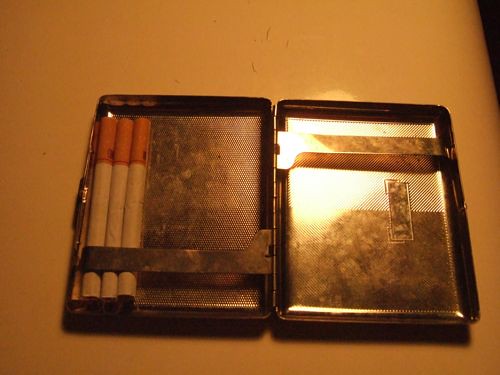In this color photograph, we see an open, vintage-looking cigarette case made of tarnished metal with a slightly rounded rectangle shape. The case, which is hinged in the middle, has a visibly worn and aged appearance, suggesting it is old and well-used. On the left side of the open case, there are three cigarettes, each with a white base and a filter that appears pinkish-brown. These cigarettes are held in place by a flat metal bar that runs horizontally across the bottom. The right side of the case mirrors the design on the left but is empty. The overall lighting in the photo is dim, giving it a gold or yellowish hue, and there is a noticeable light source shining down, reflecting off the metal surface of the right side of the case. The background of the image appears tarnished and dirty, further enhancing the vintage aesthetic of the scene.